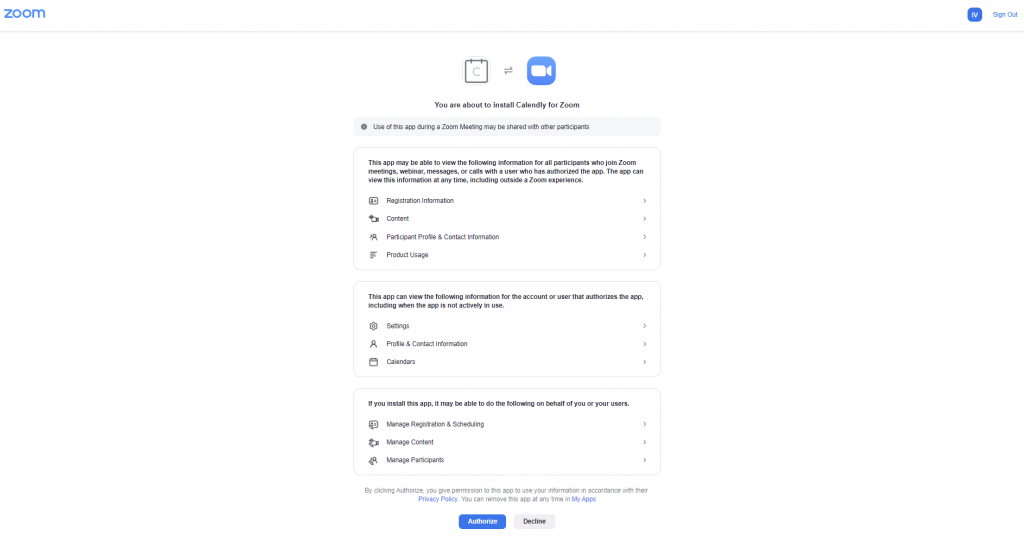The image depicts a Zoom settings page. In the upper left corner, the Zoom logo is prominently displayed in capital letters with a blue font. On the far right of the same header bar, a "Sign Out" option is visible, indicating that the user is currently logged into their account, identified by the initials "IV" in their profile icon.

The main section of the page is center-justified and organized into three distinct sections. At the top, there are three icons: a calendar icon with a "C" on it, a bidirectional arrow symbol, and a Zoom camera icon. Below these icons, a message reads: "You are about to install Calendar for Zoom." 

Following this, there's an informative bar stating, "Use of this app during a Zoom meeting may be shared with other participants," emphasizing the visibility of app usage among meeting attendees.

The page is further divided into sections for "Registration Information," "Contact," and "Product Usage," likely detailing the specifics of the app's integration and data use. At the bottom of the center-justified section are two buttons: "Authorize" and "Decline," offering the user the option to either proceed with or cancel the installation of the Calendar for Zoom app.